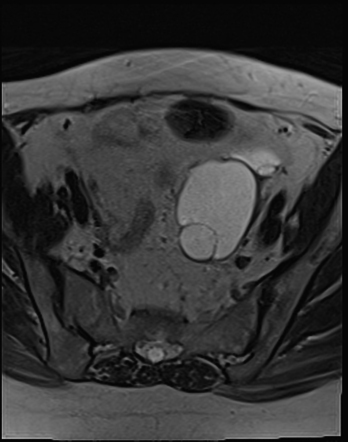This is a black and white, grayscale image that might be a high magnification of some organic structure, potentially viewed through a microscope or as an x-ray. The photograph features an assortment of irregular, circular, and oval shapes, scattered in varying shades of white, gray, and black. The central region of the image, which looks somewhat like a jumbled mass or cellular structure, is difficult to distinguish but suggests organic forms. The top of the image has a slight curvature, evoking the appearance of a hill or anatomical feature like the jaw. The background and border are solid black, emphasizing the grayscale forms in the midground. Despite its ambiguity, the image evokes the microscopic world or possibly an x-ray, with a distinctive black and white contrast.